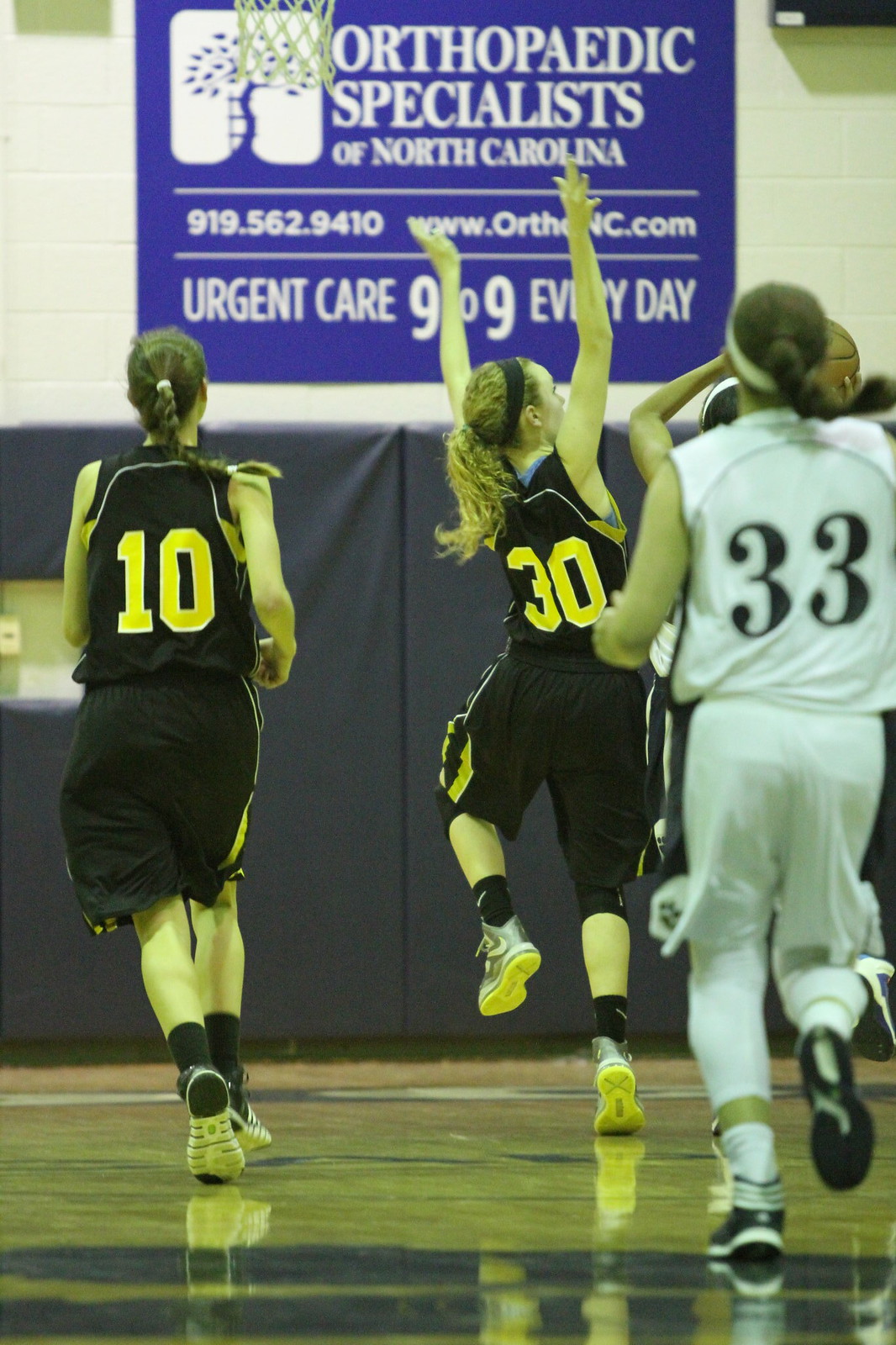In a bustling high school gymnasium, a lively girls' basketball game unfolds. The foreground reveals a dynamic scene with four players in motion. To the left, a girl in a black uniform, numbered 10 in bold yellow, is seen running. Nearby, another player in black gear, bearing the number 30, stretches her arms high, poised to block or receive a pass. Their opponent, donned in a white jersey and sporting the number 33, stands in contrast, her white leg compression stockings visible. The fourth player, partially visible, appears dark-skinned and is holding the ball, preparing for a critical shot. The court's markings are subtly seen, given the low camera angle. In the background, padded black walls ensure safety, while a prominent blue sign advertises "Orthopedic Specialists of North Carolina - Urgent Care 9-9 Every Day," emphasizing the sport's professional setting. The main colors in the image are black, white, yellow, and blue, reflecting the teams and the environment.